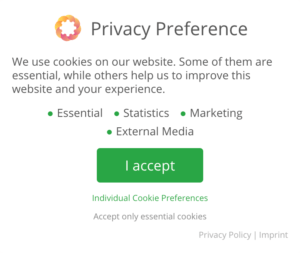This is an image featured on a website's privacy policy page. The layout consists of a clean white background with black text that reads, "Privacy Preference." The message explains, "We use cookies on our website. Some of them are essential while others help us to improve this website and your experience."

Below this explanation, there is a list titled with green dots, labeling the categories of cookies used: "Essential," "Statistics," "Marketing," and "External Media." This categorization clarifies the purposes of the cookies and their role in enhancing the website and user experience.

Beneath this list, there is a prominent rectangular button in green, with white text that says, "I Accept." Additional buttons include a green one labeled "Individual Cookie Preferences" and a purple one labeled "Accept Only Essential Cookies."

Towards the lower right area, there are two more links. One says "Privacy Policy," directing users to read the full policy, and the other says "Imprint," which could refer to the website's legal notice or a related service.

In the upper left corner of the image, near the "Privacy Preference" title, there is the website’s logo, depicted as a swirly circle featuring an orange and red color scheme.